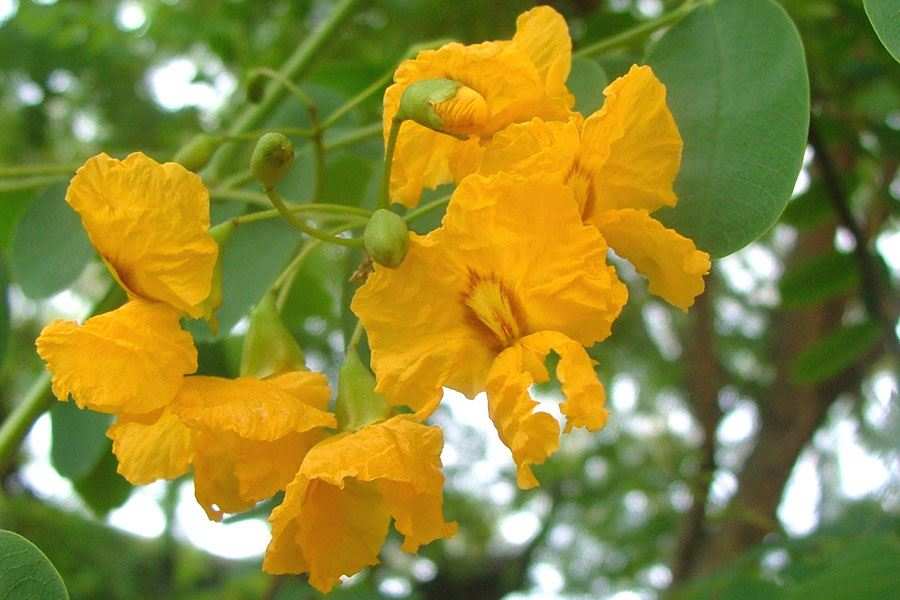The image captures a detailed outdoor scene of a yellow flower, possibly a mustard-colored or orangish-yellow shade, growing from a branch with a visible stem and surrounded by soft green leaves. It appears that the petals of the flowers are delicate and somewhat clam-shaped, with some showing signs of dryness or being wilted. The flower cluster includes various stages of growth, from unopened green buds to more mature flowers, with about two to three petals per bloom. In the background, which is out of focus, there is a tree trunk on the right-hand side along with additional foliage and a soft, white sky, suggesting an overcast day. The lighting is diffuse, creating a soft appearance without harsh shadows or direct sunlight, allowing the intricate details of the flower and its surroundings to stand out.